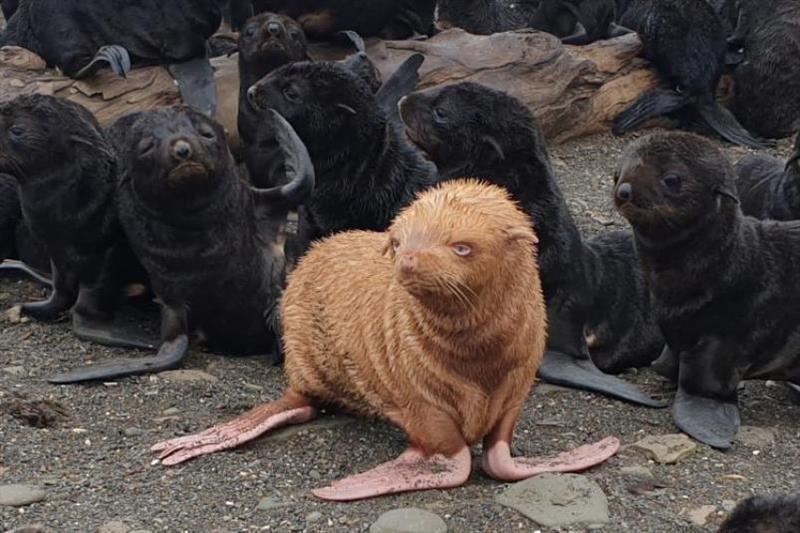In this captivating image, a group of seal pups is gathered on a gravelly shore, sprinkled with several sizable flat gray rocks. Most of the seal pups have sleek, black fur, and they are either resting on or around a long wooden log that stretches across the scene. Notably, at the forefront of this group stands a single brown seal pup, providing a striking contrast to its darker counterparts. The overall setting is a rugged, natural environment, emphasizing the stark beauty of these young marine mammals.